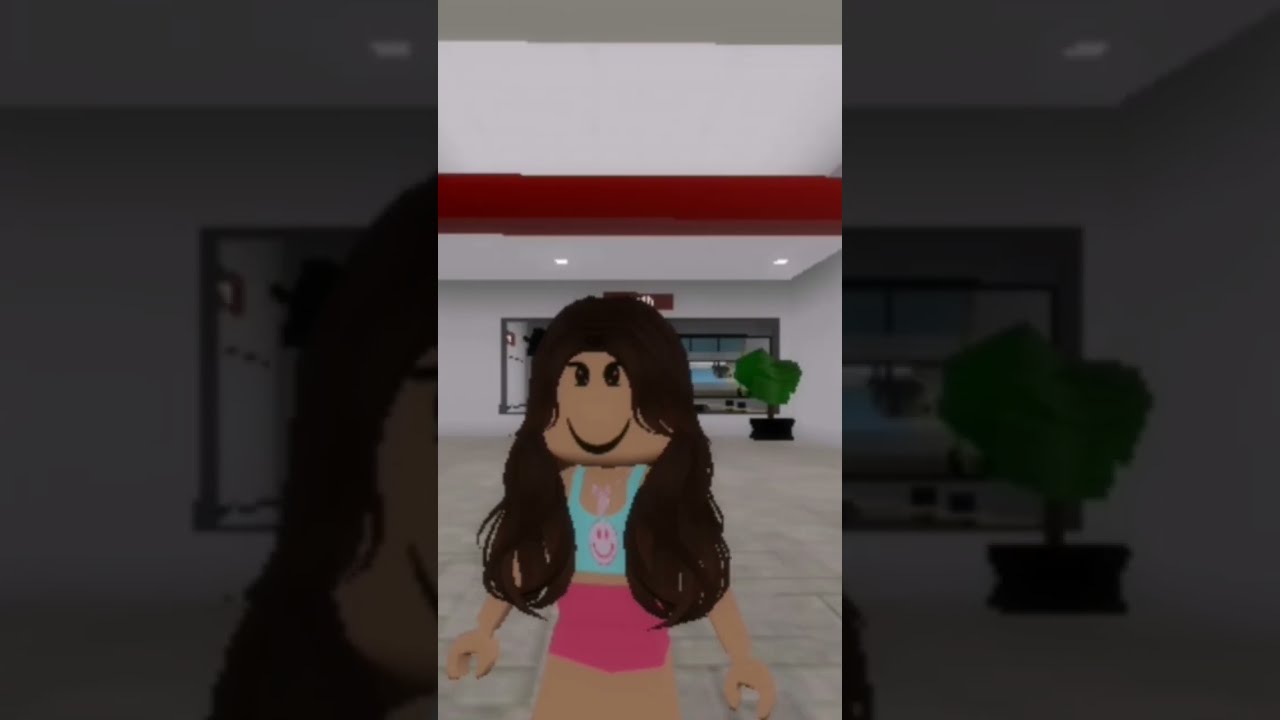The image features a crudely drawn, animated representation of a woman with long black hair and a peach complexion. She is wearing pink shorts and a light blue tank top adorned with a pink smiley face. Her facial features include big, beady black eyes and a simple smile. The character’s form is somewhat reminiscent of a Lego figure, with a large, square head, a big blob-like shape for legs, and U-shaped hands.

In the background, there is a white and red wall with a ceiling above, accentuated by a digital window. Behind her left shoulder stands a potted tree with a black stand, a brown base, and typical green leaves. The overall setting and style suggest a piece of crudely drawn artwork, possibly created digitally.